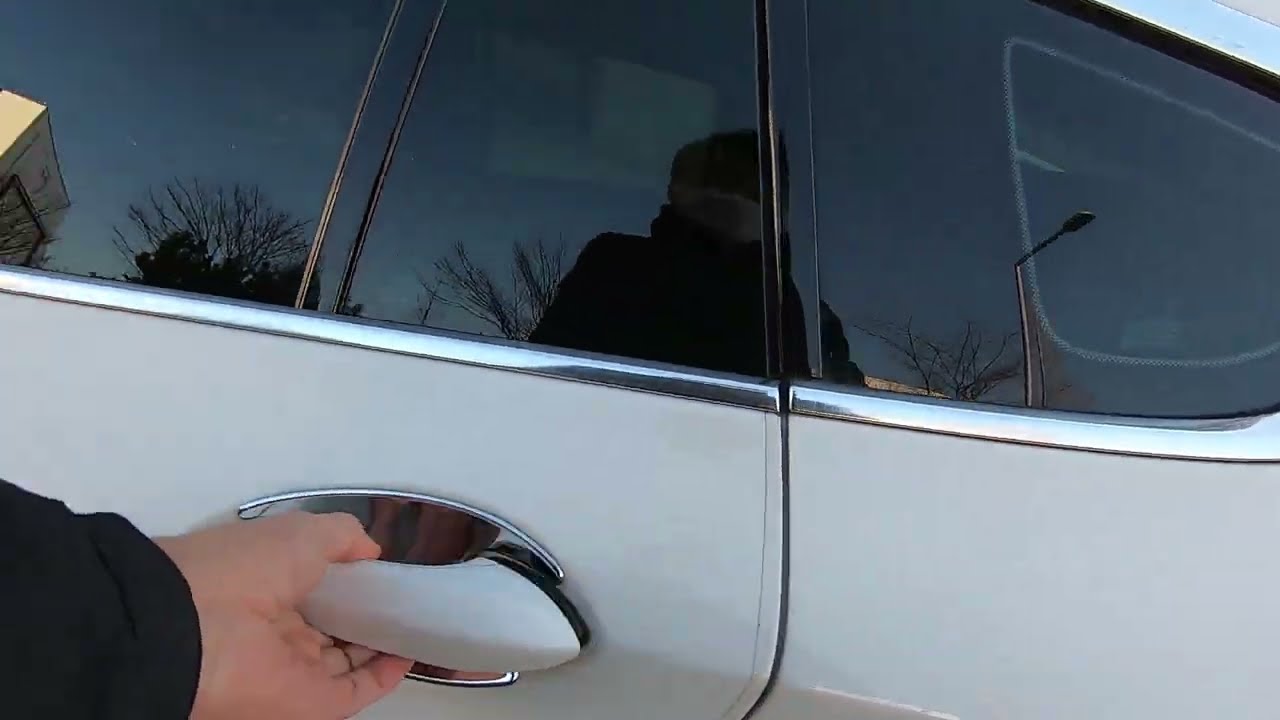In this image, an individual is preparing to open a rear passenger-side car door of an off-white, pearl-colored vehicle. The car features black tinted windows accented with a chrome frame. The person, whose left hand is seen gripping the door handle, is dressed in a black long-sleeve jacket and a hat, and their reflection in the car's window also shows they are wearing a medical mask. The background reflection in the car's windows includes multiple trees—some with leaves and others barren—suggesting it might be winter. Additionally, a white building and a distinctive L-shaped light pole are visible in the reflection, contributing to the outdoor setting of the scene.